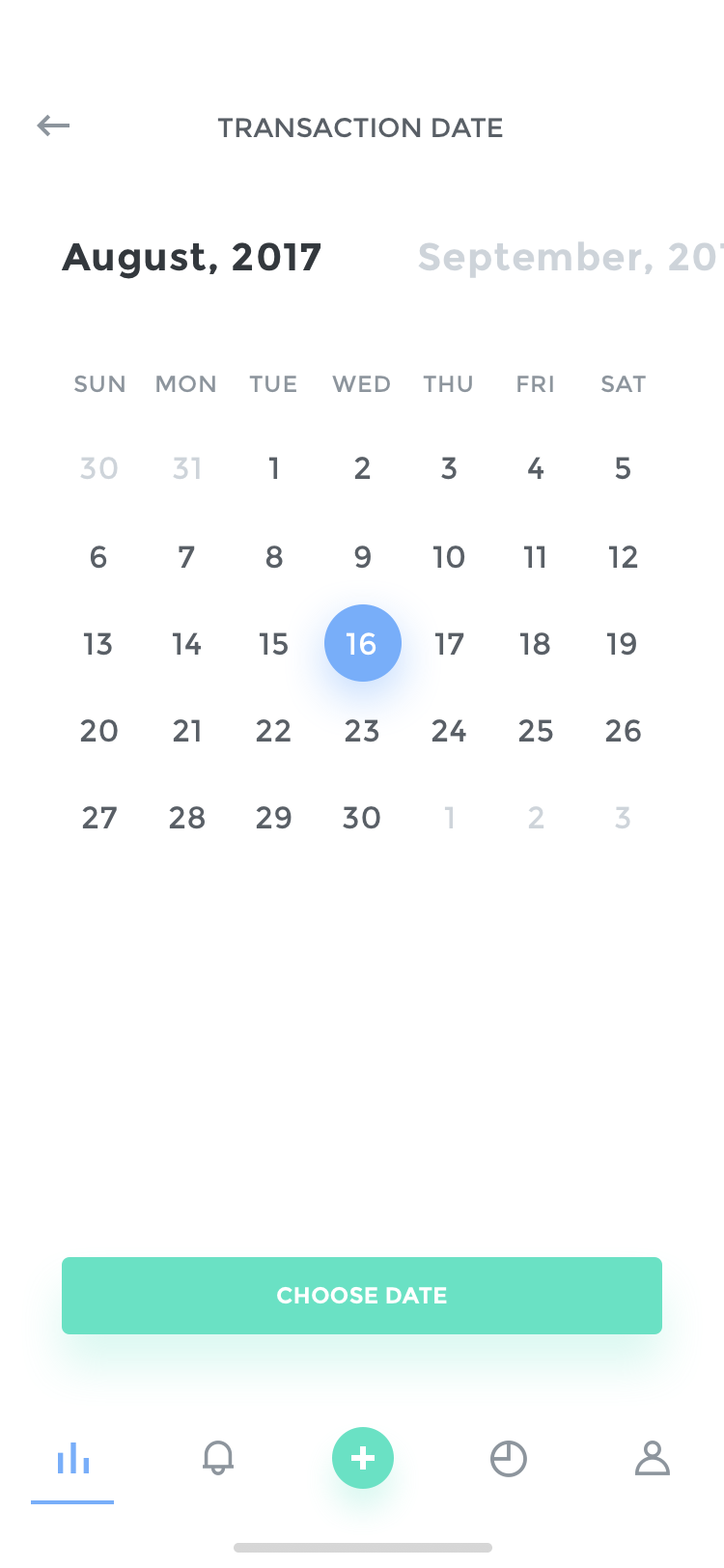In the image, a digital calendar interface is displayed prominently. At the top of the screen, the title "Transaction Date" is centered, with a left arrow icon positioned just to its left. Beneath the title, "August 2017" is highlighted, while "September 2017" appears in gray to the right, indicating it as the next selectable month.

The calendar layout follows, starting from Sunday on the left and proceeding to Saturday on the right. The month of August 2017 begins on a Tuesday and concludes on Wednesday the 30th. A blue circle highlights the date Wednesday, August 16th. 

Below the calendar, there is a turquoise rectangular button with the label "Choose Date" in white text. 

At the bottom of the screen, five icons are aligned horizontally: 
1. A graph icon on the far left.
2. A notification bell icon.
3. A turquoise circle featuring a plus sign in the center.
4. A clock icon.
5. A profile silhouette icon on the far right.

The entire interface is set against a clean, white background.